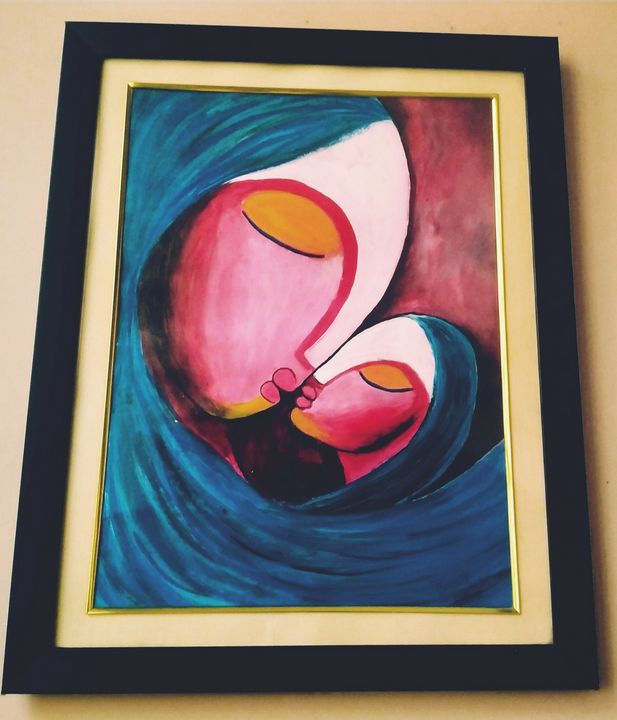This is a color photograph of a painting, captured in a detailed setting that appears to be indoors, as the painting is seen hanging on a tan, beige-painted wall. The painting is encased in a dark brown frame with a light brown matting that adds a layer of sophistication and contrast.

The painting itself features a stylized portrayal of a woman with long, flowing blue hair that sweeps dramatically across her shoulders in sweeping, curved lines reminiscent of the letter "C." Her hair, vibrant and wavy, sets a striking contrast to the vivid colors of her face. The woman's face is distinctly red with white on her forehead, except for her eyes, which are set in an oval field of red, giving her an intense, expressive gaze. Her features include red cheeks, orange eyebrows, subtle eyelashes, and two vividly red lips. She leans tenderly towards a child who mirrors her appearance. The child, looking up at the woman while the woman gazes down, shares the same long blue hair, red lips, red cheeks, and white forehead, creating a cohesive visual bond between them.

In the top right-hand corner of the painting, there is a striking red area that balances the vibrant color scheme of the figures below. The image itself does not contain any text, allowing the viewer to focus purely on the abstract, emotive interaction between the two figures and the bold, whimsical use of color and line.